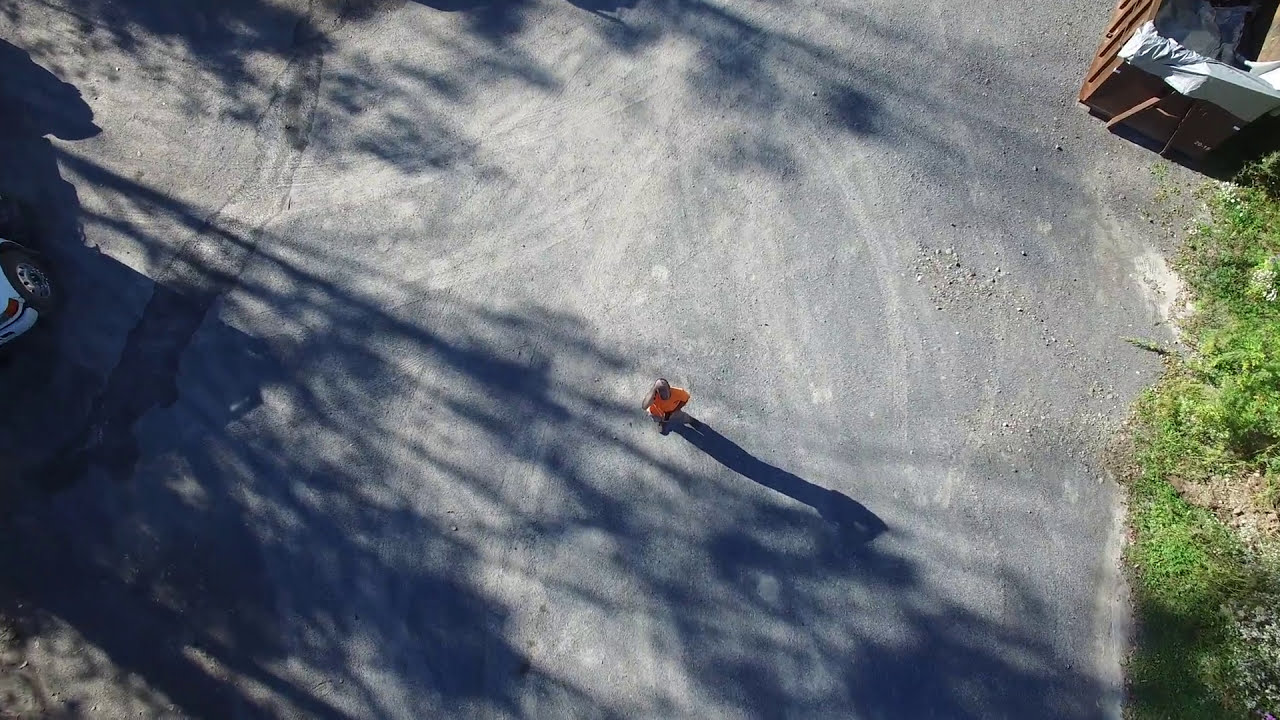This overhead photograph captures a solitary man standing in the middle of a large, gravelly, gray area that resembles an unfinished driveway or concrete surface with tire marks. The man, wearing an orange t-shirt and possibly blue jeans, is looking up at the camera with his hand shielding his eyes from the sun. Shadows from off-picture trees extend across the gravelly ground to the left. In the upper right corner of the image, there's a large brown industrial dumpster, while the bottom right shows a touch of greenery with some green bushes. Additionally, the left side of the image partially reveals the rear bumper and one tire of a white car.